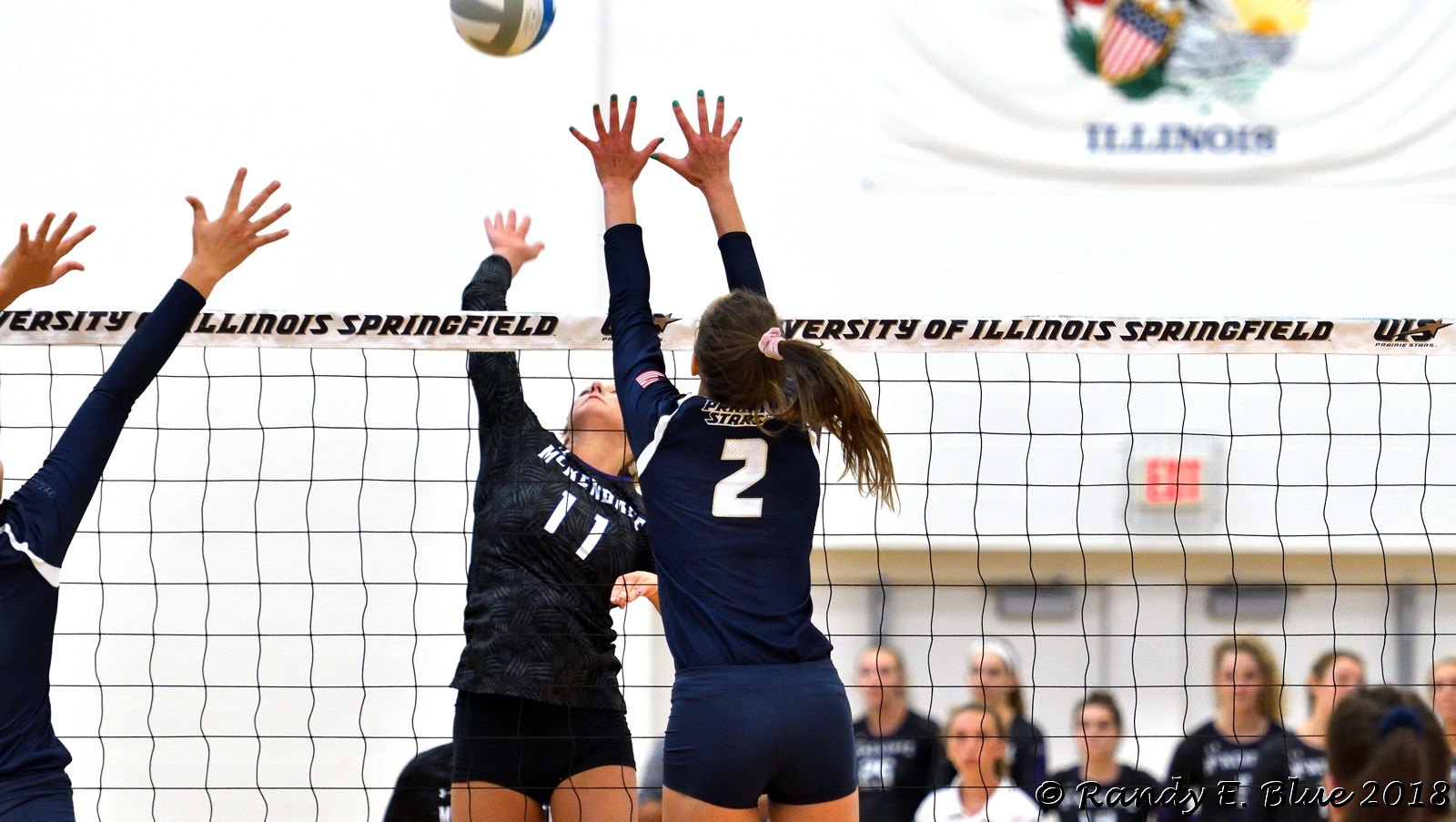The image captures a dynamic moment in a college women's volleyball match between the University of Illinois Springfield and an opposing team. At the center of the photo, a player in a blue jersey with the number 2 leaps with her hands raised, preparing to spike the blue and white volleyball that hovers just above her fingertips. Opposite her, an opponent in a black and gray-striped jersey with the number 11, also airborne, extends her hands in an attempt to block the spike. A teammate on the left side, partially off-screen, also has her hands up, moving diagonally to support the block. The bright, white-lit gymnasium features a prominent "Illinois" flag and the University of Illinois Springfield name displayed on the top of the net. Spectators are seen watching intently below the flag, while the room's brightness is accentuated. The photo, dated 2018, bears the copyright of Randy E. Blue in the lower right corner.